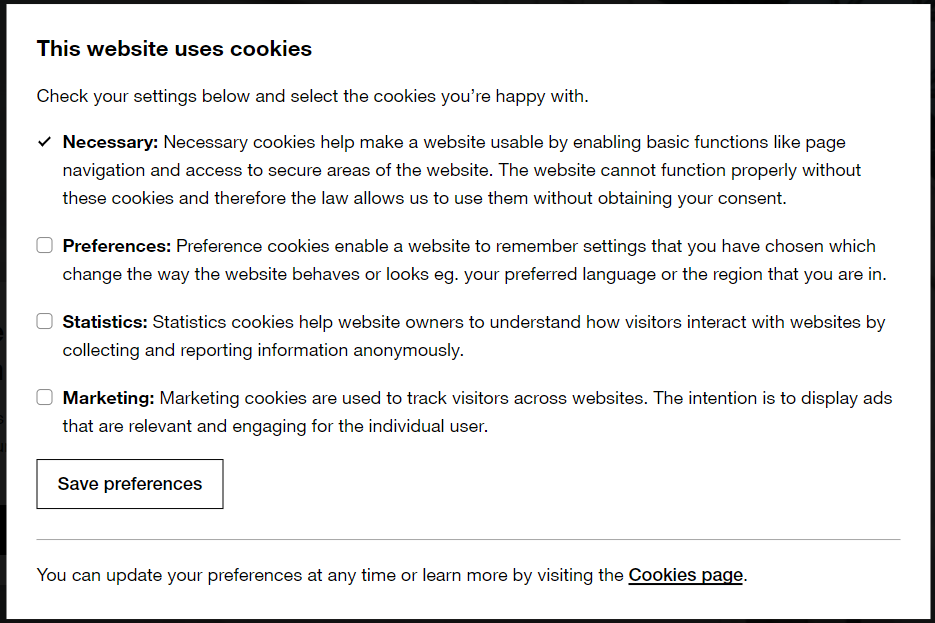This image is a screenshot from an unidentified webpage featuring a cookies consent banner. The banner is displayed in black text on a white background, encapsulated by a thin black border. The message informs users that the website uses cookies and prompts them to adjust their settings accordingly. 

The text states, "This website uses cookies. Check your settings below and select the cookies you're happy with." It then lists various types of cookies:

1. **Necessary**: This option is pre-selected. Necessary cookies make the website usable by enabling basic functions like page navigation and access to secure areas. These cookies are essential for the website's proper functioning and are used without requiring user consent.
   
2. **Preferences**: These cookies allow the website to remember user settings, like preferred language or regional settings, altering its behavior or appearance.
   
3. **Statistics**: These cookies collect and report anonymous data to help website owners understand visitor interactions and improve user experience.
   
4. **Marketing**: Marketing cookies track visitors across different websites to display ads that are more relevant and engaging for individual users.

The banner concludes with options to "Save preferences" and a reminder that users can update their preferences anytime or learn more by visiting the cookies page. The image is strictly text-based, void of any photographs, illustrations, people, animals, or plant life.